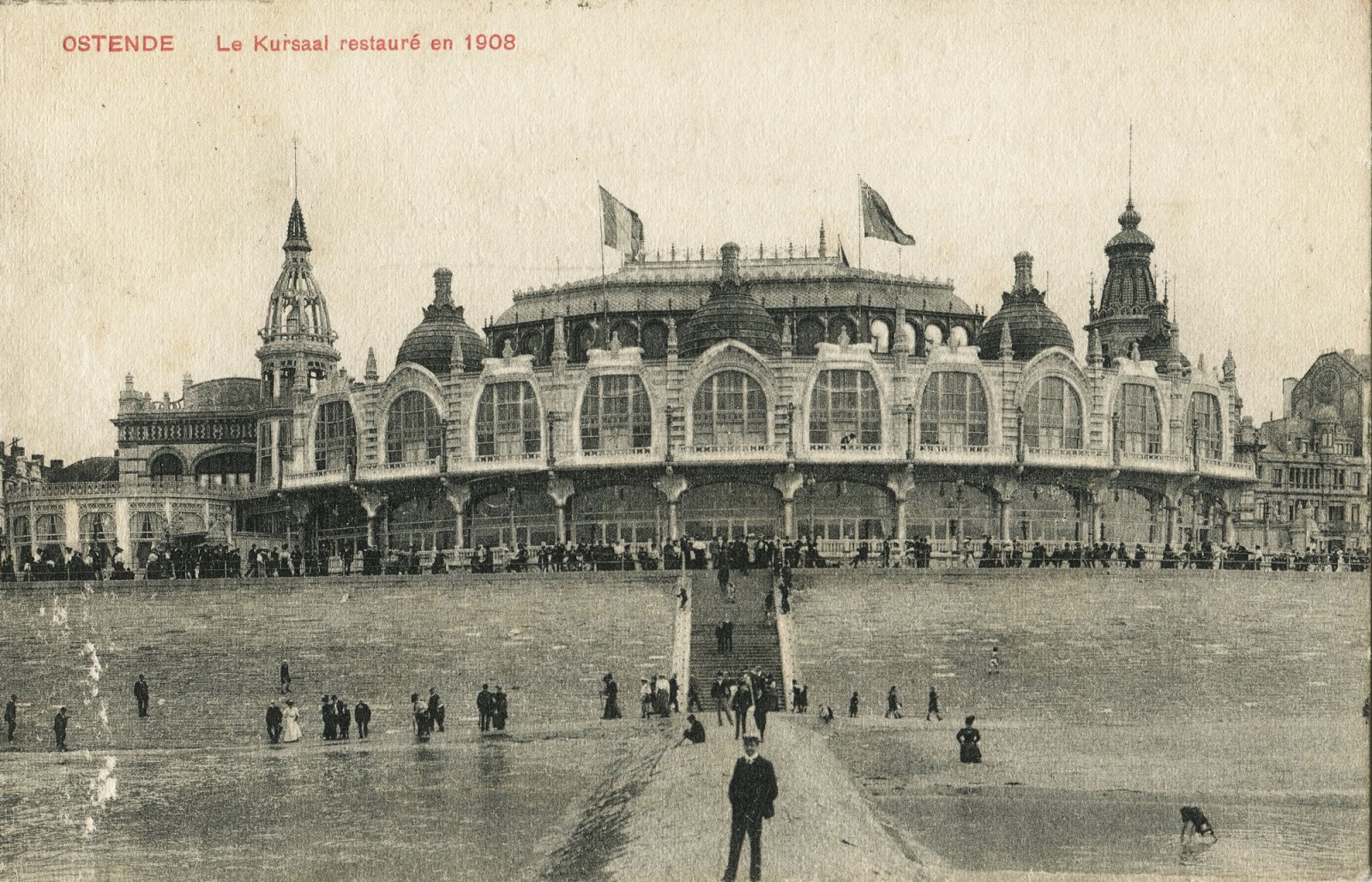This is a very detailed black-and-white photograph from 1908, indicated by red text in the top left that reads “OSTENDE” in bold, all caps, and “LA CURSAL RESTAURANT” with mixed capitalization. The image captures a grand, historic building known for its partially circular, curved facade adorned with numerous, large arched windows. The building stands majestically atop a hill, accessible by a central path with sloping sides leading to a staircase. On either side of this raised sand walkway, you can see children playing by the water, suggesting the building is on a waterfront or beach.

The structure itself appears to be two or three stories high, with the second floor slightly larger and supported by multiple pillars and columns. Two large flagpoles, each hoisting a flag, are posted on the roof. The building is also capped with crenellated domes from which spires jut out. The photograph showcases a large number of individuals, likely more than 50, gathered in front of the building on the sloping lawn or grassy area. Among these people is a single gentleman in a suit and hat in the foreground, though his features are indistinct due to the distance from the camera. This well-preserved image provides a glimpse into early 20th-century architecture and social gatherings.